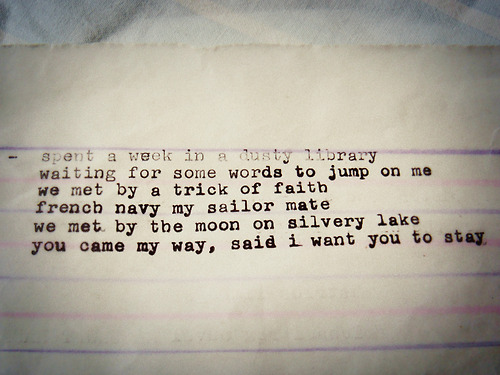This image captures a well-worn piece of lined paper, slightly crumpled and showing signs of wear at the top, suggesting it may have been wet or crinkled. The paper is placed on a light blue blanket or sheet. The page is lined with widely spaced blue and pink lines, although some lines appear to be a darker purple. In the center of the page, there is typewritten text in black ink, and it reads: "spent a week in a dusty library, waiting for some words to jump on me, we met by a trick of faith, French Navy, my sailor mate, we met by the moon on Silver Lake, you came my way, said I want you to stay." Notably, the 'I' is not capitalized, adding a personal touch to the typed message.